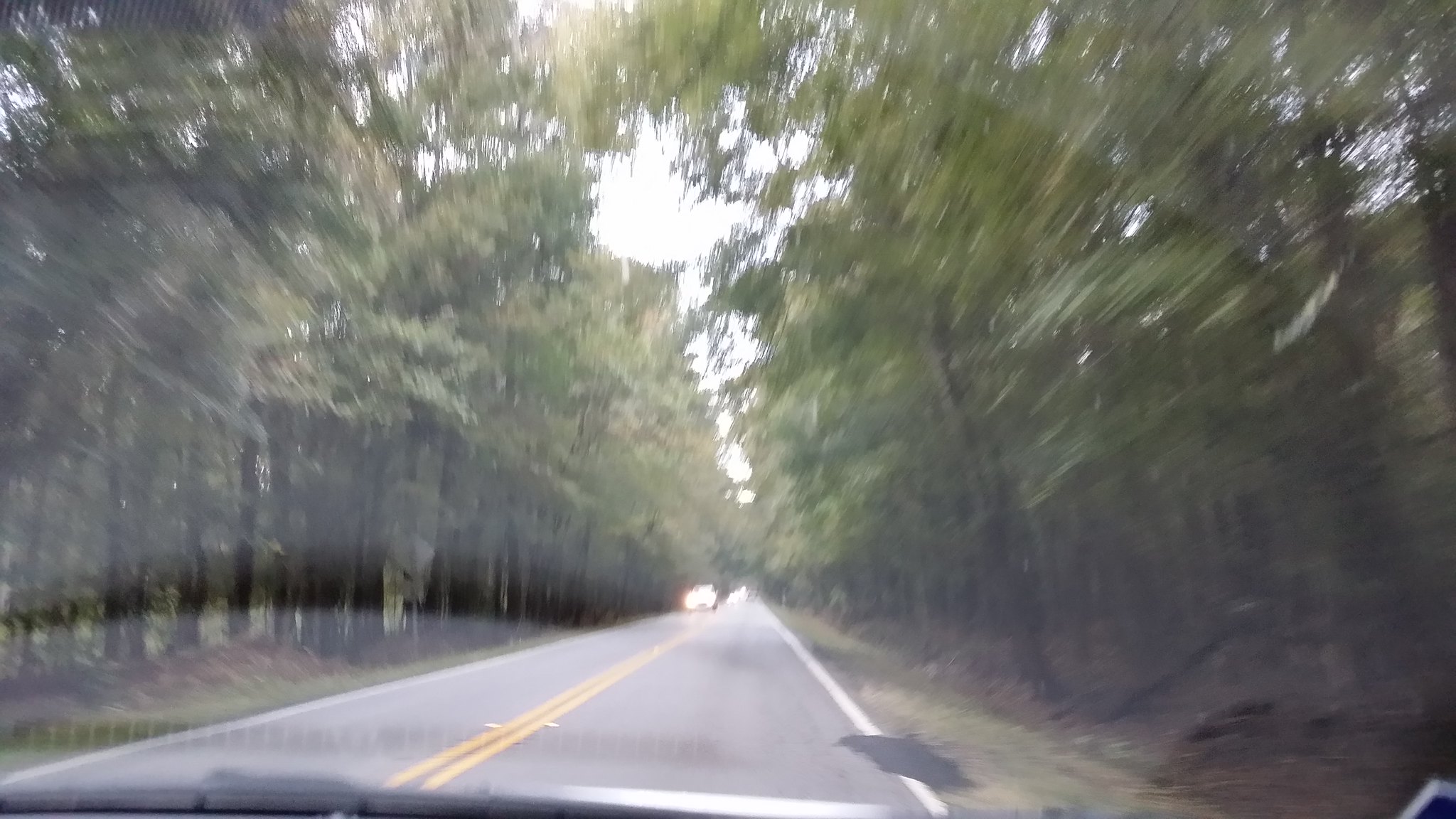The digital photo captures a scenic daytime view through the windshield of a moving car. The photograph, taken in landscape mode, reveals a stretch of lighter black asphalt road flanked by tall trees with brown trunks and lush green foliage high above. The road is marked by solid white lines on each side and a double yellow center line, which appears to narrow as it extends toward the horizon. On the right side of the road, a patch of darker asphalt indicates a repaired section. In the bottom left corner, the black windshield wiper of the car is visible, while the upper right portion of the windshield shows a slightly dirtier area. There’s a patch of whitish dirt that hasn’t been cleaned. Farther down the road, headlights from an oncoming car are discernible but indistinct. The atmosphere is bright, with a whitish-blue sky peeking through the tall trees, suggesting a sunny day.